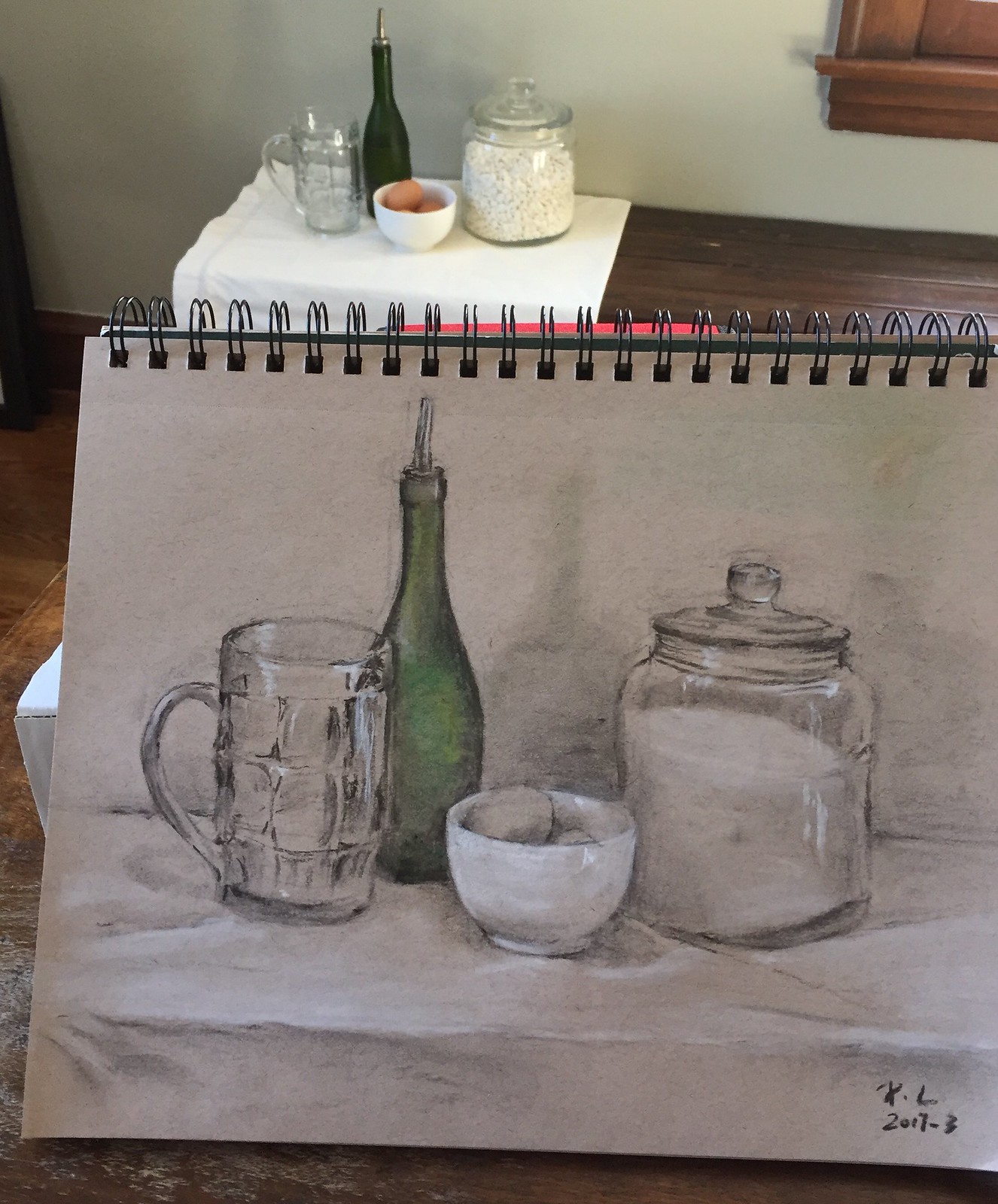In this evocative photograph, an artist can be seen meticulously painting a still life of a table setting directly in front of him or her. The table, set in a rustic setting, features a brown wooden surface adorned with a pristine white cloth. At the far left, a white bowl cradles a collection of brown eggs, exuding a simple yet elegant charm. Just to the left of the bowl stands a distinctively dimpled, empty mug. Adjacent to these items is a slender oil bottle, possibly intended for olive oil, and a jar filled with what appears to be rice, or perhaps white candy, adding texture and variety to the scene.

The top right-hand corner of the photograph reveals a brown wooden window sill and frame, adding a warm, homey backdrop to the composition. The artist holds up their sketch pad at an angle, aligning it with the actual table setting, creating a layered visual effect wherein art imitates life. The sketch pad bears a detailed drawing of the setup, signed "K.L." and dated March 2007, showcasing the artist's dedication and the date of their creative endeavor. This photograph beautifully captures the intimate process of art-making, highlighting both the serene simplicity of the subject and the artist’s focused engagement with their work.